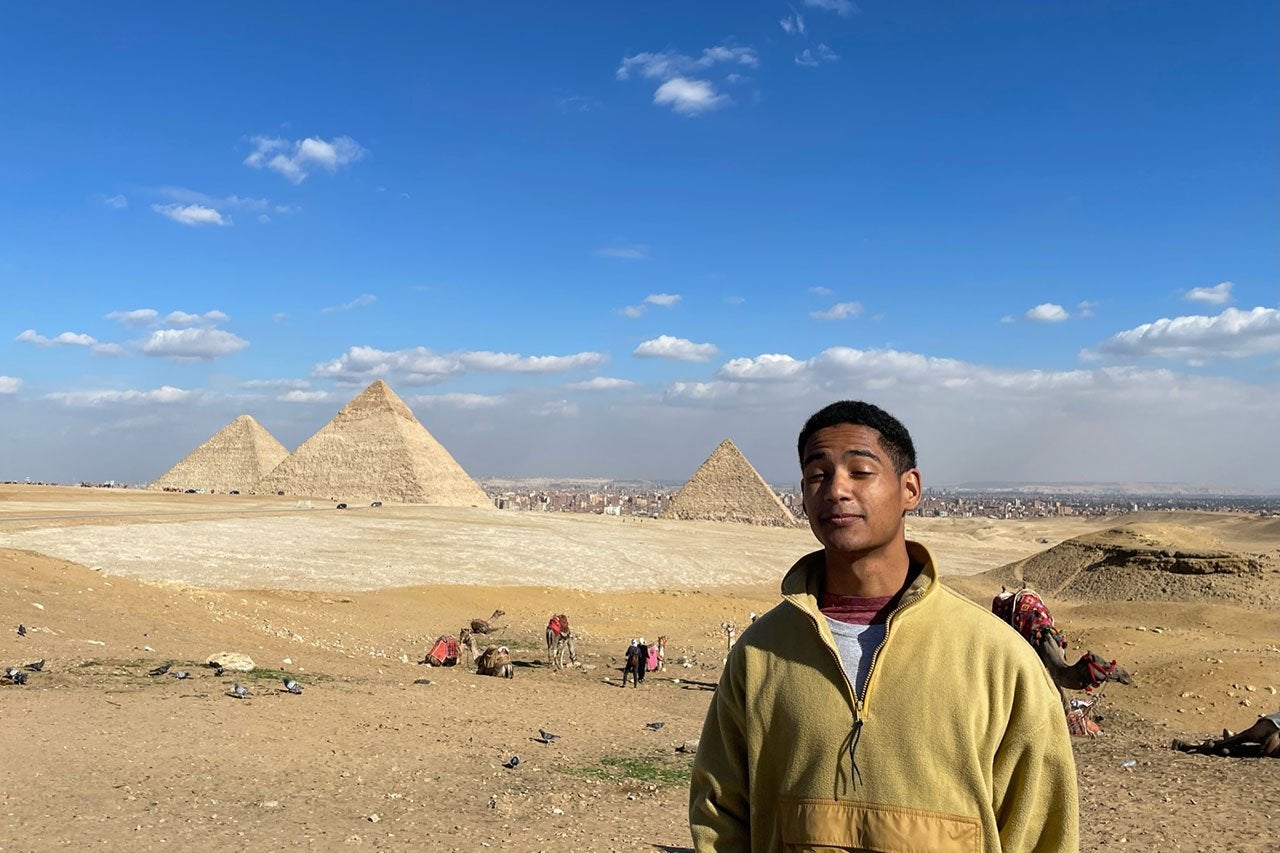This photograph captures a striking scene of the pyramids at Giza with the sprawling city of Cairo visible in the far distance behind them. The three pyramids are centrally positioned against a backdrop of a blue sky dotted with white, fluffy clouds. The sandy landscape stretches out in the foreground, where a gentleman stands prominently from waist up. He is a black man, wearing a dingy yellow zip-up hoodie with a bemused smile on his face and his eyes closed. To his right, a camel is resting on the ground, while to his left, in the distance, there are five more camels adorned with various fabrics and what seems to be luggage. The image is not a selfie, suggesting someone else took the photo, capturing the gentleman as he stands before the iconic pyramids. There are also some people scattered in the background, adding more life to this historic and picturesque scene.